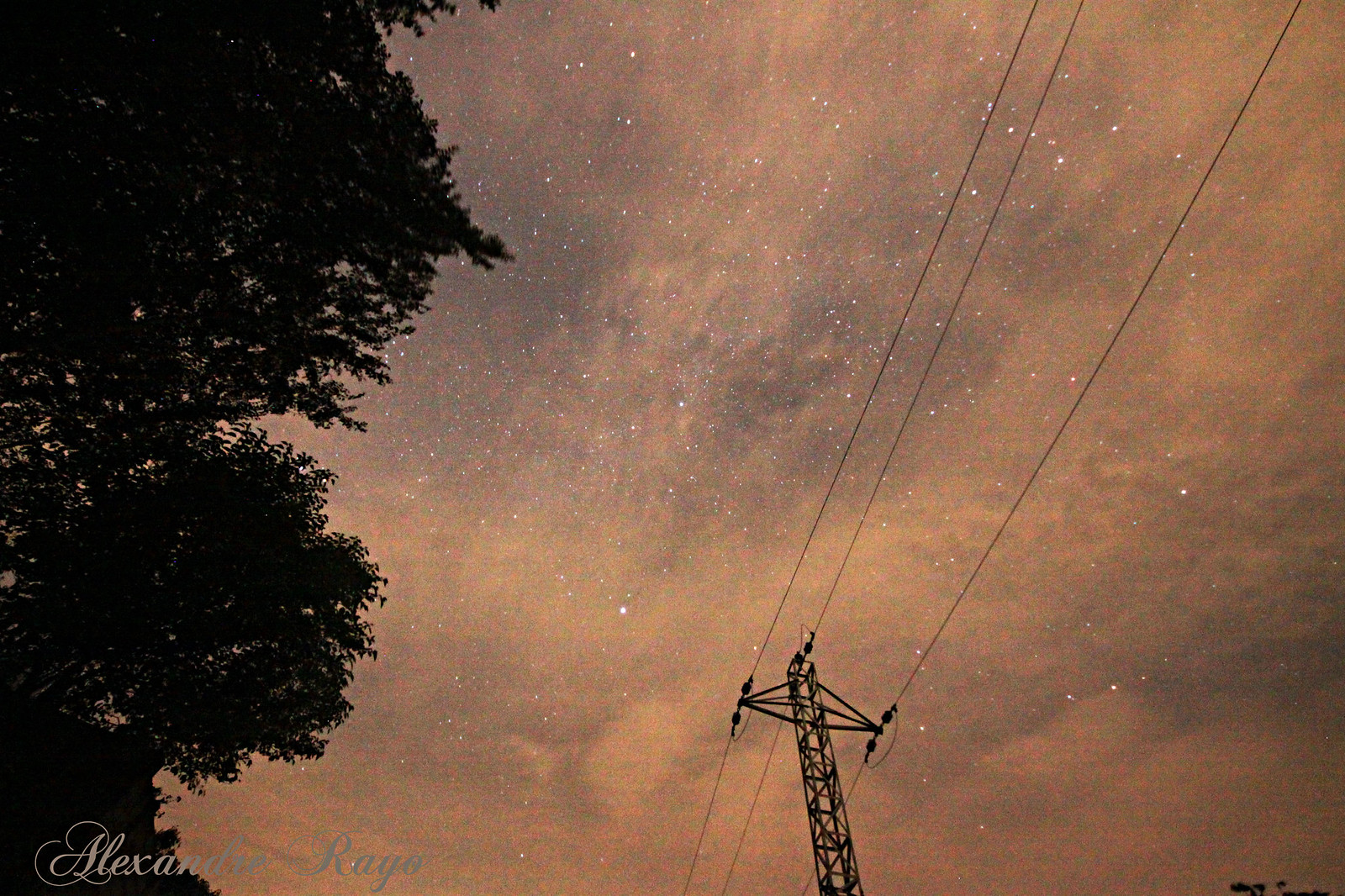This image captures a serene evening sky transitioning to night, with a hazy, grayish backdrop tinged with dusty reds and subtle pinkish-white clouds. The sky is filled with faint, twinkling stars emerging through the thin cloud cover. Dominating the right side of the photograph is a tall, dark metal utility pole with three power lines extending outward—one to the left, one to the right, and one upwards. On the left edge of the image, dark silhouetted treetops stretch from the top to the bottom, creating a stark contrast against the sky. At the bottom left corner, the name "Alexander Real" is inscribed, adding a personal touch to this enchanting twilight scene.